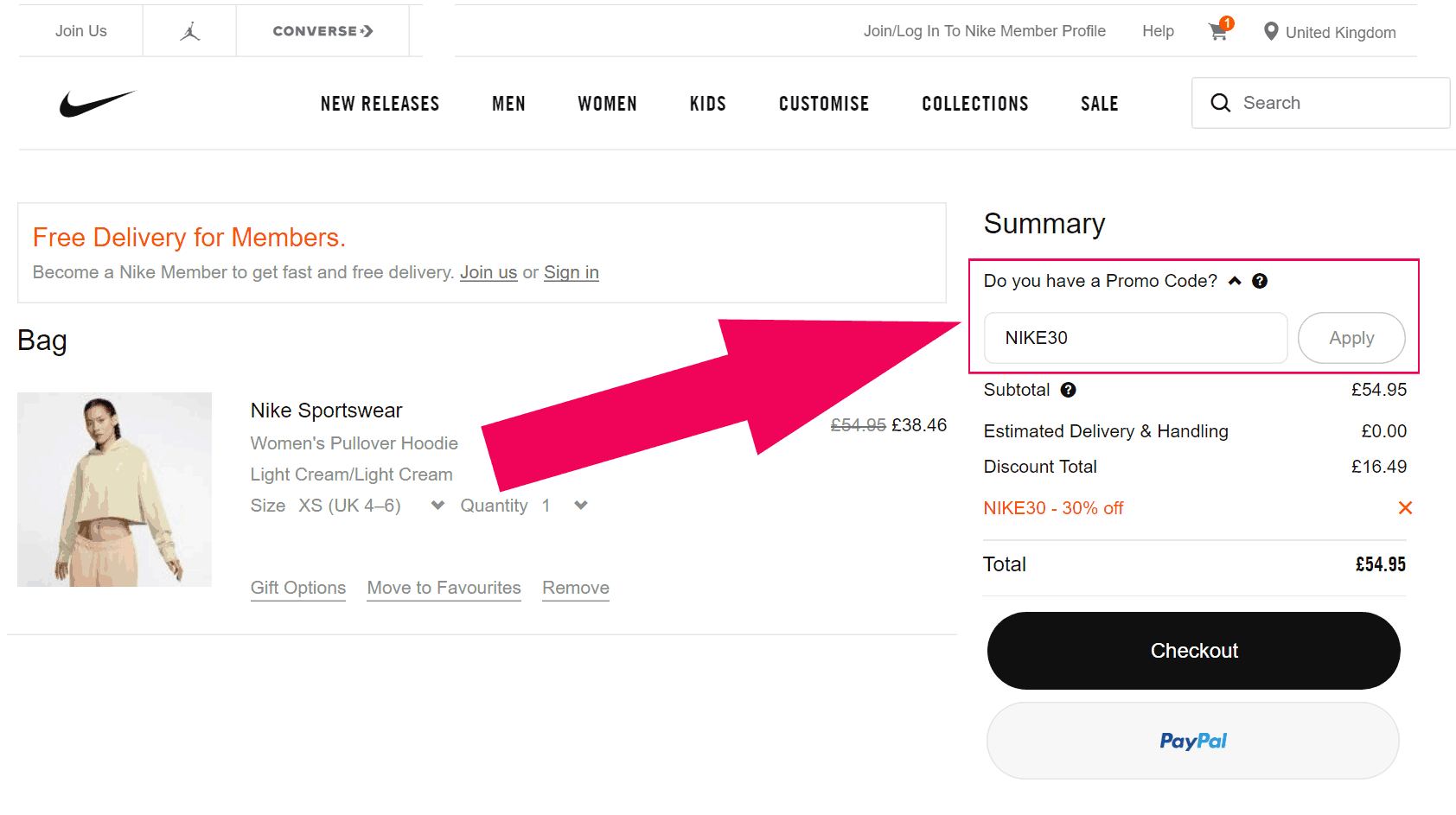On the Nike website's cart section, labeled "Bag," lies a detailed display of a single item: a Nike Women's Pullover Hoodie from the Nike Sportswear collection. The item is in a light cream color and is sized extra small (UK size 4-6). The quantity is specified as one. Below the item details, there are options to add gift packaging, move the item to favorites, or remove it from the cart.

Dominating the screen is a large red arrow pointing to the promo code section, which currently has "NIKE30" entered, applicable by clicking the button on the right of the box. The subtotal for the item is listed as £54.95, with no delivery and handling fees. The promo code "NIKE30" provides a discount of £16.49, bringing the final total to £54.95. The site prominently mentions a special offer: free delivery for members, encouraging users to sign up or sign in to take advantage of fast and free shipping.

A picture of a Caucasian woman wearing the light cream pullover hoodie accompanies the item details. The top of the webpage features navigation links to other sections, including "New Releases," "Men," "Women," "Kids," "Customized," "Collections," and "Sale."